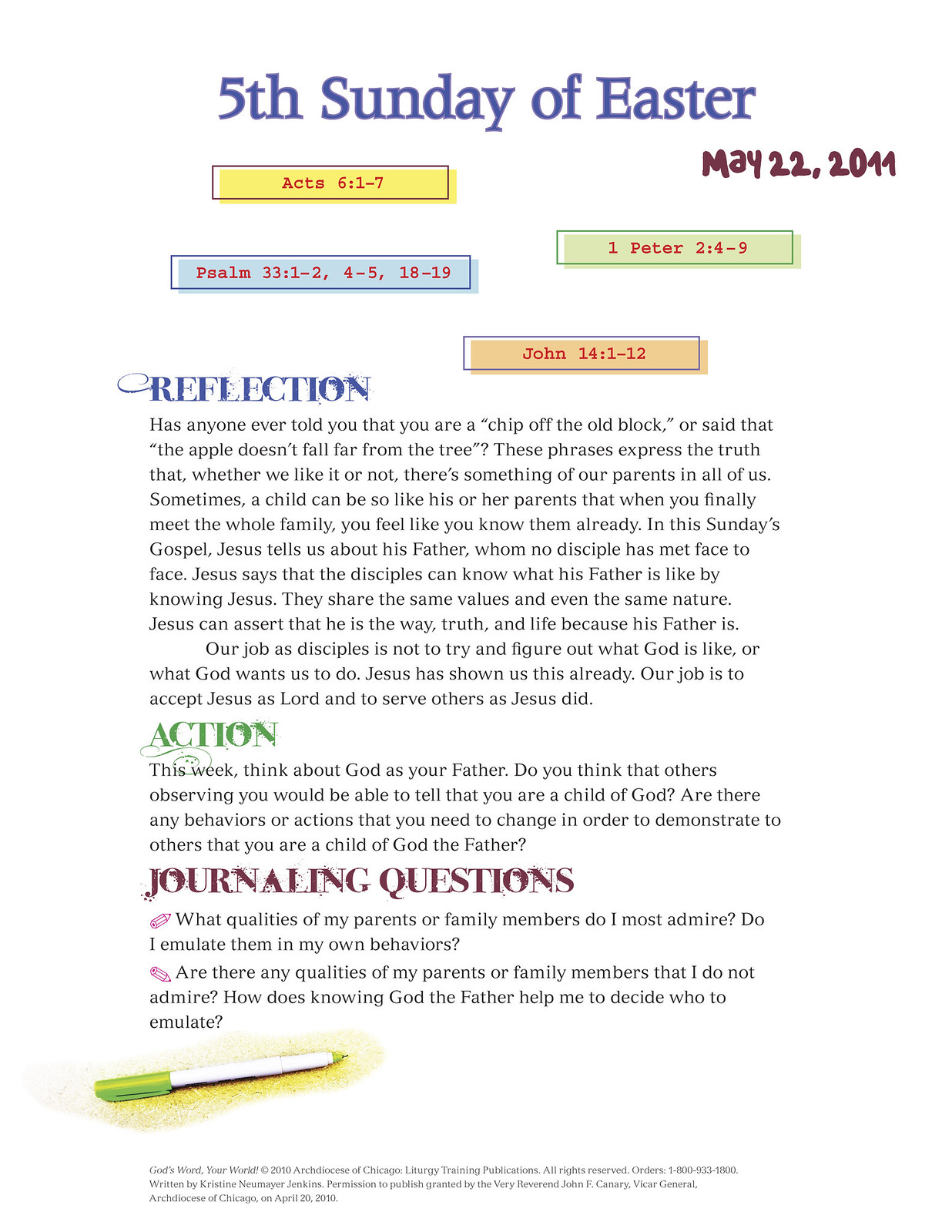The image depicts a scanned piece of paper with a white background, prominently titled in blue lettering as "5th Sunday of Easter." Adjacent to this title, in the upper-right corner, is the date "May 22, 2011" written in burgundy. Beneath the title and date, the page is sectioned into several rectangles, each in distinct colors with red text. The first rectangle is yellow, listing "Acts 6:1-7," followed by a blue rectangle with "Psalm 33:1-2, 4-5, 18-19." To the right of these, a green rectangle indicates "1 Peter 2:4-9," and beneath all these is an orange rectangle specifying "John 14:1-12."

Below these scripture references, the content is divided into three sections with headers: "Reflection" in blue, "Action" in green, and "Journaling Questions" in burgundy. The "Reflection" section includes a detailed paragraph emphasizing the idea that we inherit traits from our parents and drawing parallels to knowing God the Father through Jesus. The "Action" section encourages readers to contemplate how their behavior reflects their identity as a child of God. The "Journaling Questions" section prompts two reflective questions: one about admiring and emulating family qualities, and the other concerning qualities less admired and how one's understanding of God influences these perceptions. At the bottom of the page, there is an image of a white pen with a green cap and tip.